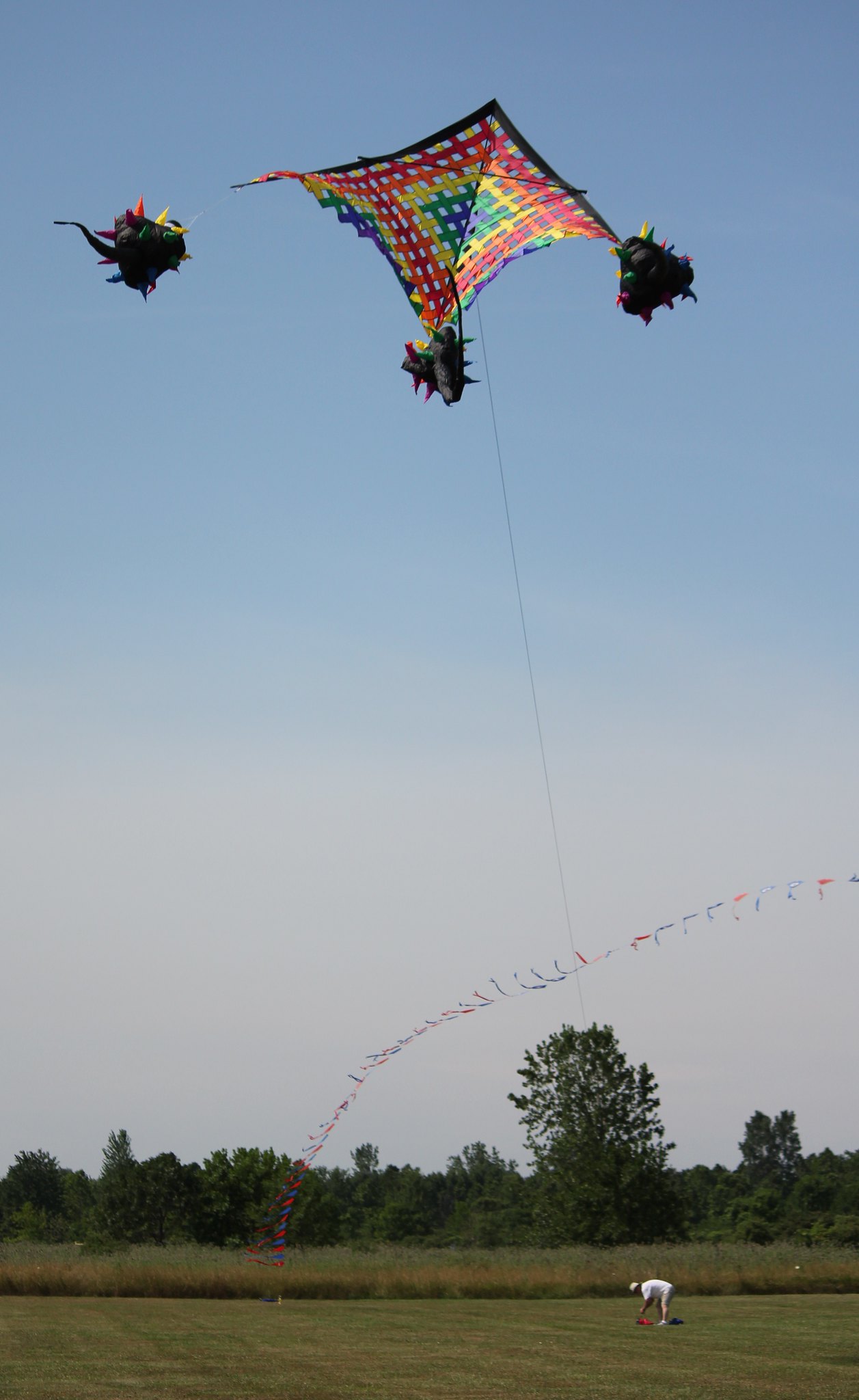The image captures a vibrant scene of a wide grassy field leading into a backdrop of green bushes and tall trees under a sky transitioning from a dull blue at the top to a whitish hue near the horizon. In the middle of the field, a small figure, dressed in a white shirt and a hat, is bending down, appearing to handle a large, intricate kite. The kite, the focal point of the image, is an impressively large diamond shape adorned with a crisscrossed pattern in a spectrum of colors including red, yellow, blue, green, orange, and a purplish-blue. Suspended from the kite are three dark, spiky objects that resemble mythical creatures, each decorated with colorful horns matching the kite's palette. Above the man, a long string extends skyward, adorned with blue and red banners fluttering in the breeze. This lively scene blends elements of nature with the playful, artistic spectacle of kite flying.